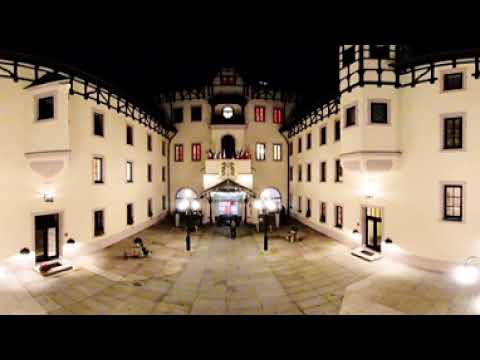This photograph, captured at night, features a sizable, cream-colored European building spanning the entire frame. The building stands three stories tall with black accents and a detailed architectural design. The structure's symmetry is evident, with both the left and right sides adorned with various windows—some illuminated, others dark. Four windows in the middle section exhibit a distinctive reddish tint, likely due to curtains behind them. The building's lower portion is marked by several doors and windows, leading to a stone-paved entrance area. The top of the building is crowned with intricate gating-like detailing running across its width. A courtyard with street lamps can be seen, emphasizing the nighttime setting as all exterior lights are turned on. Notably, the image is devoid of any people and displays a slight lens distortion.